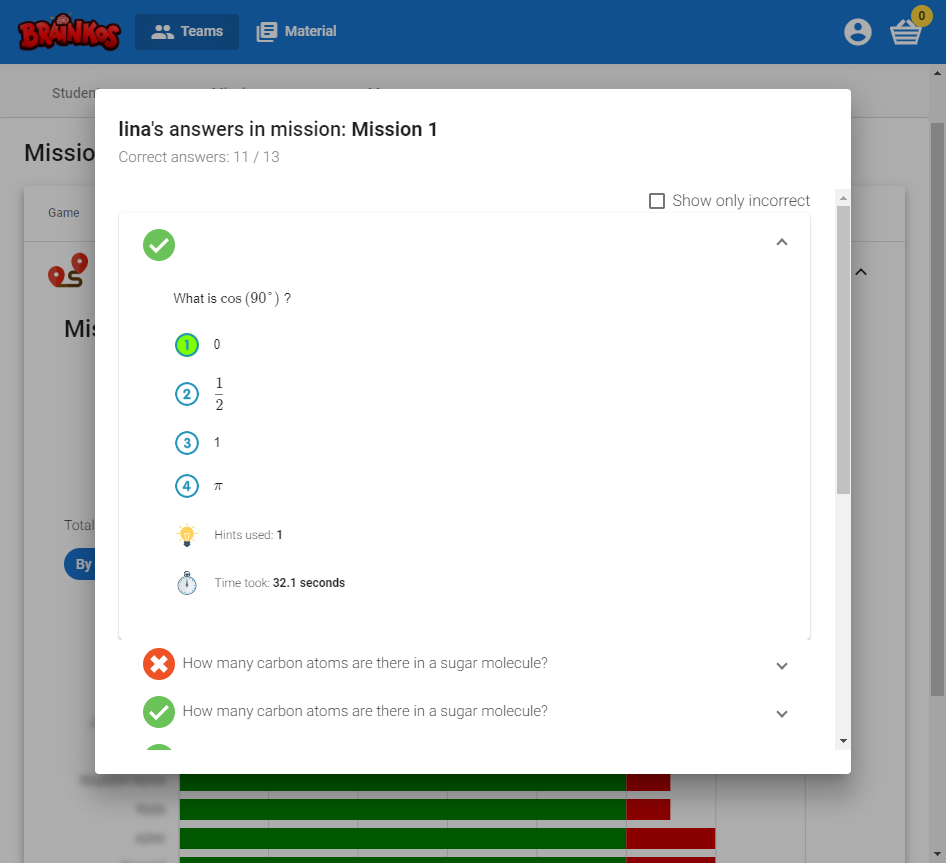A screenshot captures a pop-up on a website, with the background page darkened and a blue header at the top. To the left of the header is a child-like red logo with a dark red outline that reads "BRAINCOS," with a brain icon serving as the dot on the "I". Next to it, within a dark blue rectangle with rounded corners, is a white icon of two people and the text "TEAMS". Further right, there is a white icon of a double-sheeted paper, followed by the text "MATERIAL." On the top right corner of the header, there's a round white profile picture icon and a white shopping basket icon with a yellow circle housing a black zero.

Below the header, the body of the darkened web page is visible with a white background. Central to this is a pop-up with rounded corners and a white background. The pop-up's title at the top left, in bold black text, reads "LENA'S ANSWERS IN MISSION: MISSION 1." Below this, light gray text aligned to the left states "CORRECT ANSWERS 11 / 13." Towards the bottom right of the pop-up, medium gray text next to a medium gray checkbox reads "SHOW ONLY CORRECT." Underneath this, a thin light gray line outlines the first question, which starts in the top left with a green circle containing a white checkmark, followed by the question text.